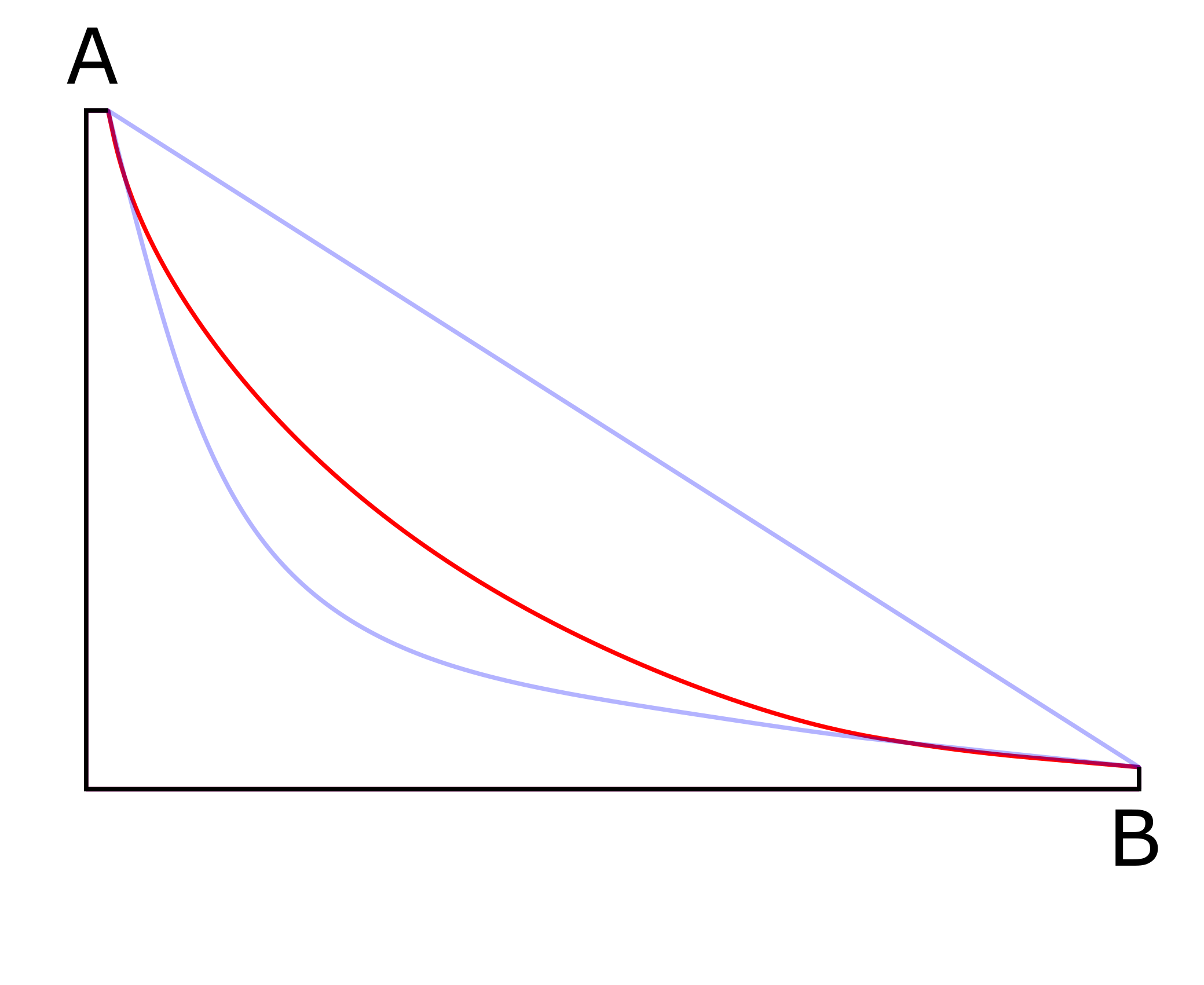The image depicts a graphical chart set against a clear white background. It features an X and Y-axis type layout with a vertical line, labeled 'A' in a capital letter at the top left corner, and a horizontal line labeled 'B' at the bottom right corner. Attached at the intersection of these axes, there is a longer horizontal line extending fully across the chart, ending with a short upward tick. 

There are three distinct lines that connect point A to point B. The first is a light purple curved line, the second is a red curved line positioned slightly above the purple one, and the third is a straight diagonal purple line that runs directly from A to B. The straight purple line represents a direct path, while the red and light purple lines represent different curvature paths, resembling Brachistochrone curves. Each element is clearly defined, ensuring the chart's structure and layout are easily understood.